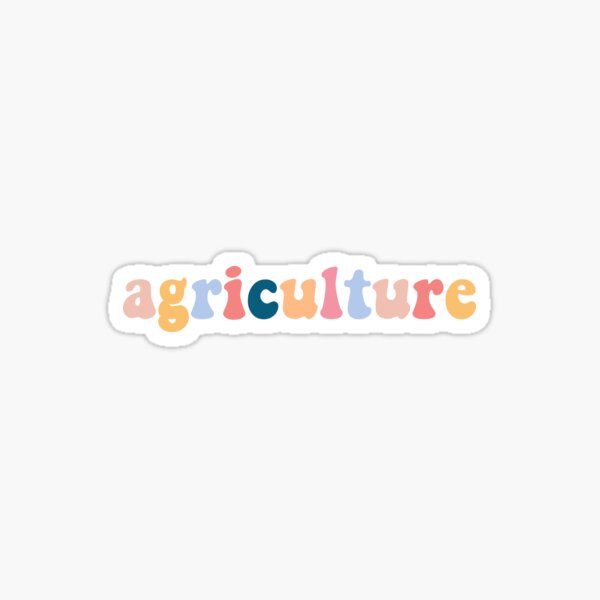The image features the word "agriculture" displayed in lowercase, multicolored bubble letters. Each letter is distinct in color: the 'A' is pink, the 'G' is orange, the 'R' is light blue, the 'I' is dark pink, the 'C' is dark blue, the 'U' is coral, the 'L' is purple, the 'T' is light blue, the second 'U' is pink, the second 'R' is dark pink, and the 'E' is orange. The letters are set against a white backdrop specifically shaped to the contours of the word, making it stand out. This white shape is outlined by a squiggly gray line which further separates it from the overall light gray background. The font style is reminiscent of a playful, bubbly, hippie aesthetic, adding to the image's vibrant and lively feel.